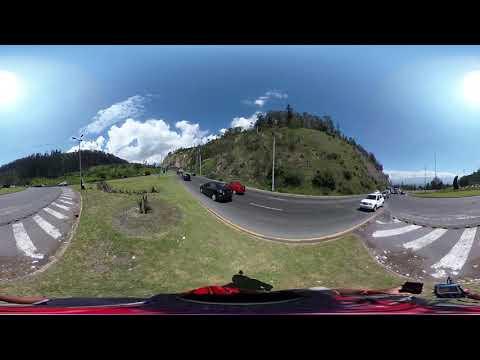In this panoramic image, a blue sky with white clouds stretches across the top, bordered by a thick black line. Half of the sun can be seen on both the left and right sides. Dominating the foreground is a big, faded green hill with scattered bushes and short trees. The hill is partly bare, revealing patches of dirt. Surrounding this hill is a semicircular road that continues straight to the right; it features white stripes and a roundabout. Cars populate the road, including black, red, and white vehicles in various positions. A white car is visible on the right side near a turning point, flanked by a black and red car side by side. The road itself is lined with light posts, and another gray road with white stripes loops around the hill. In the image, you can also notice a patch of gray with white stripes on the left, and some red detail towards the front. Further back, beyond the central hill, other smaller hills covered in vegetation and a small mountain with many trees can be seen. The entire base of the image is bordered by a thick black line.